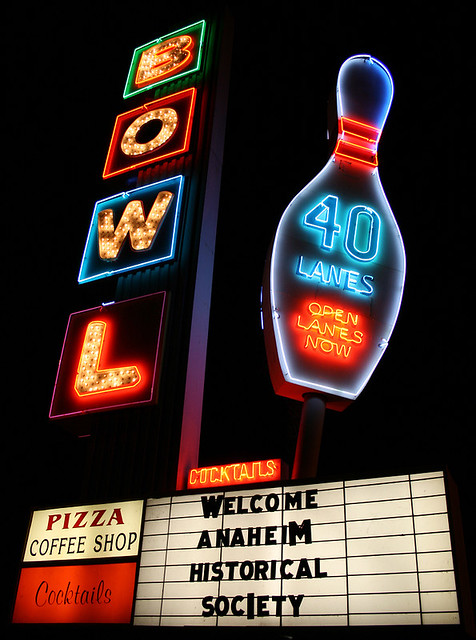This vertical night-time photograph captures an illuminated bowling alley sign. Dominating the left side, the neon letters "B-O-W-L" run vertically down what appears to be a pole or the side of a building. Adjacent to this, on the right, is a large neon bowling pin highlighted in white with red stripes, which reads "40 lanes, open lanes now." At the base of the image, there are multiple signs: a white letter board featuring the message "Welcome Anaheim Historical Society," and two smaller signs to its left indicating "Pizza Coffee Shop" and "Cocktails." The main colors in the image are shades of black, white, orange, blue, red, and purple, making the neon signage vividly pop against the night sky. A lighter, reflective pillar with colorful accents partially frames the scene, contributing to the vibrant, inviting ambiance of this vintage bowling alley.